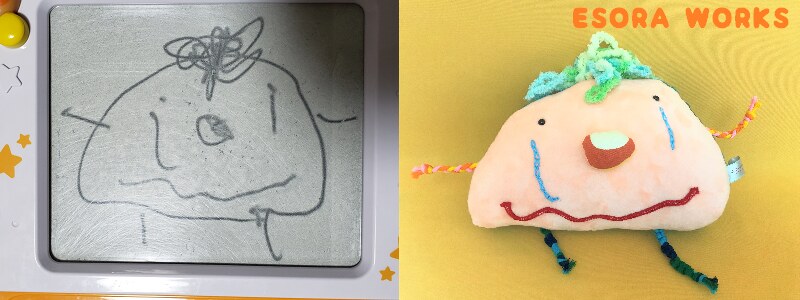The image features two distinct but related visuals. On the left, there's a mostly black and gray pencil or Etch-A-Sketch drawing of a quirky, humanoid figure. This figure has an exaggerated, round head with tiny arms extending from where the ears might be and little legs protruding from where the jaw would normally be. Its facial features are minimalist, adorned with small blue dots for eyes from which blue teardrops stream downward, a button nose, and a squiggly red line serving as a smile. The frame encasing this sketch is white and decorated with yellow stars and a white star.

On the right side, there is a colorful rendition of the same figure. This figure is crafted to look like a plush toy, primarily comprised of a large, pale flesh-toned head with similar blue teardrop lines beneath its eyes, an orange and white nose, and a long red stripe for a mouth. Its hair is a textured tangle of green, blue, and yellow yarn. The figure's legs are depicted with a patchwork of blue, black, and green fabric. Above the colorful figure, the text "Isora Works" (spelled E-S-O-R-A) is prominently displayed. The overall composition draws a playful comparison between the monochrome sketch and the vividly colored plush figure, emphasizing their whimsical, almost melancholic expressions.